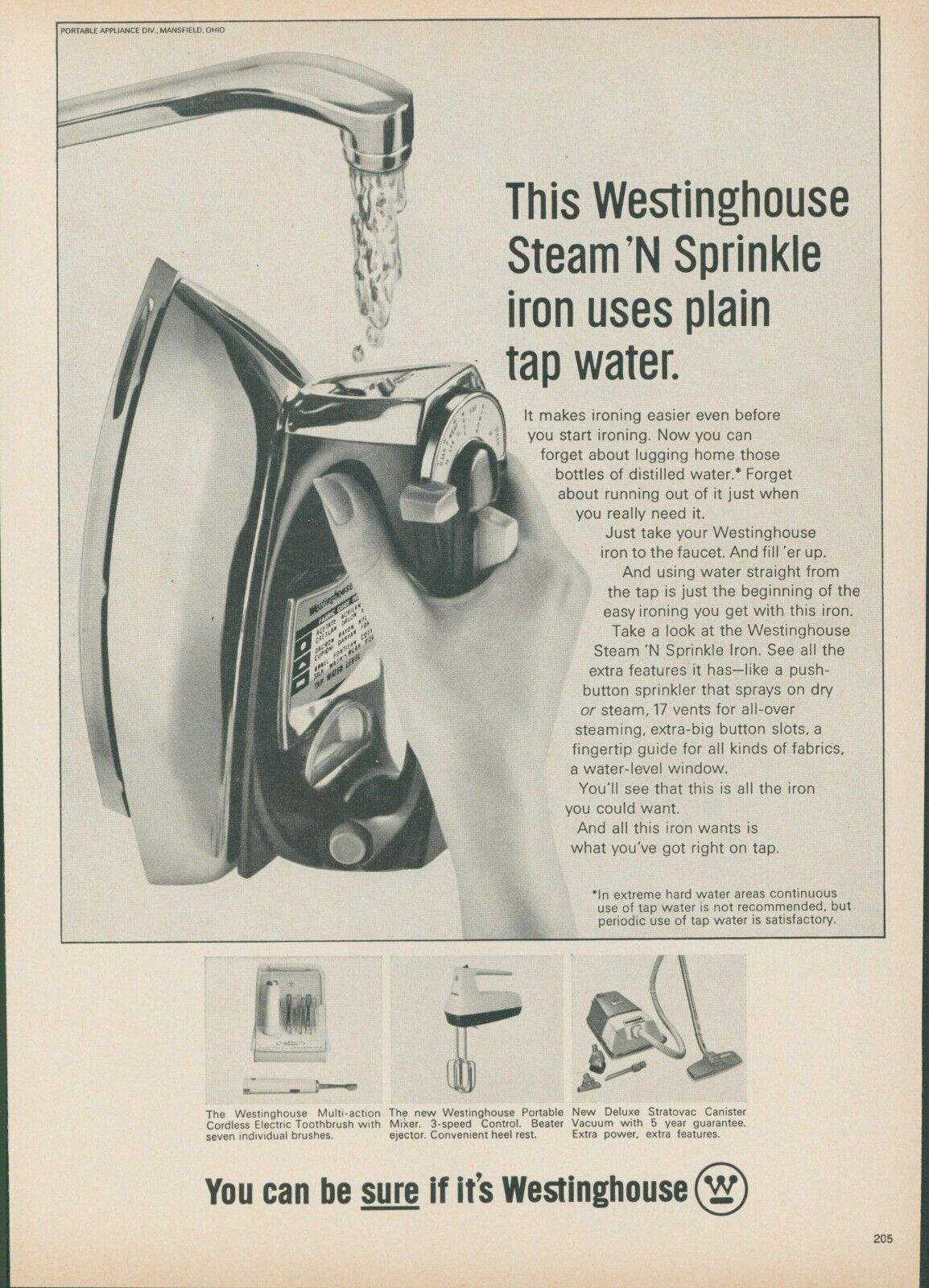The image is a vintage black-and-white advertisement for the Westinghouse Steam and Sprinkle Iron, featured on page 205 of a magazine. A woman’s hand is pictured holding the iron under a water faucet, from which water pours directly onto the iron, emphasizing its use of plain tap water. The headline reads, "This Westinghouse Steam and Sprinkle Iron uses plain tap water," highlighting its convenience. The advertisement extols the benefits of no longer needing to buy distilled water—just fill the iron right from the tap. Additional features of the iron include a push-button sprinkler for both dry and steam functions, 17 vents for uniform steaming, extra-large button slots, a fingertip guide for various fabrics, and a water level window. The page also displays images of other devices like a handheld blender, a portable vacuum cleaner, and an electric toothbrush. The Westinghouse logo, a “W” with a line under it, is prominently featured along with the tagline, "You can be sure if it's Westinghouse," reinforcing the brand’s reliability. Overall, the iron promises to make ironing easier even before starting, with all essential features readily evident in the visual layout.